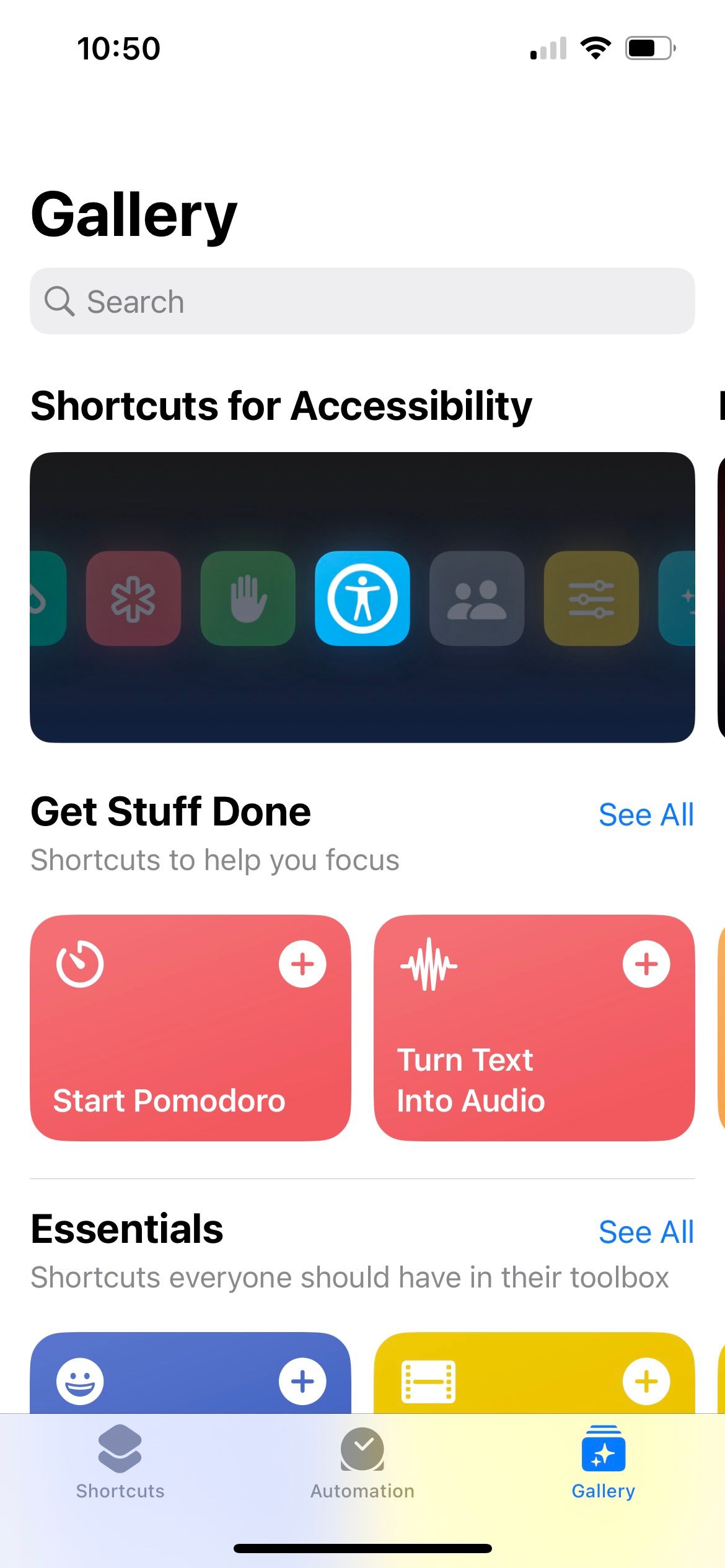This is a screenshot of a smartphone interface with a white background. In the top left corner, the time is displayed as 10:50 in black text. The top right corner shows three icons: a network signal indicator, a Wi-Fi signal icon, and a battery icon, all in black. Below the time, the word "Gallery" is written in black, accompanied by a search box labeled "Search." Underneath the search box, a text reads "Shortcuts for accessibility."

A series of icons is displayed next. First, a blue and white accessibility shortcut icon, followed by a white and green pan icon, an icon depicting two people, and an orange settings icon. Beneath these icons, the text "Get stuff done, shortcuts to help you forecast" is written. A blue button labeled "See all" is positioned below this text.

At the bottom, there are two red buttons labeled "Pomodoro" and "Turn text to audio." The bottom section features the text "Essential shortcuts everyone should have in their toolbox," accompanied by blue and yellow icons on the left and right, respectively. Finally, three navigation buttons are positioned at the very bottom: "Shortcuts," "Automation," and "Gallery." The "Gallery" button is highlighted in blue, while "Shortcuts" and "Automation" are gray.